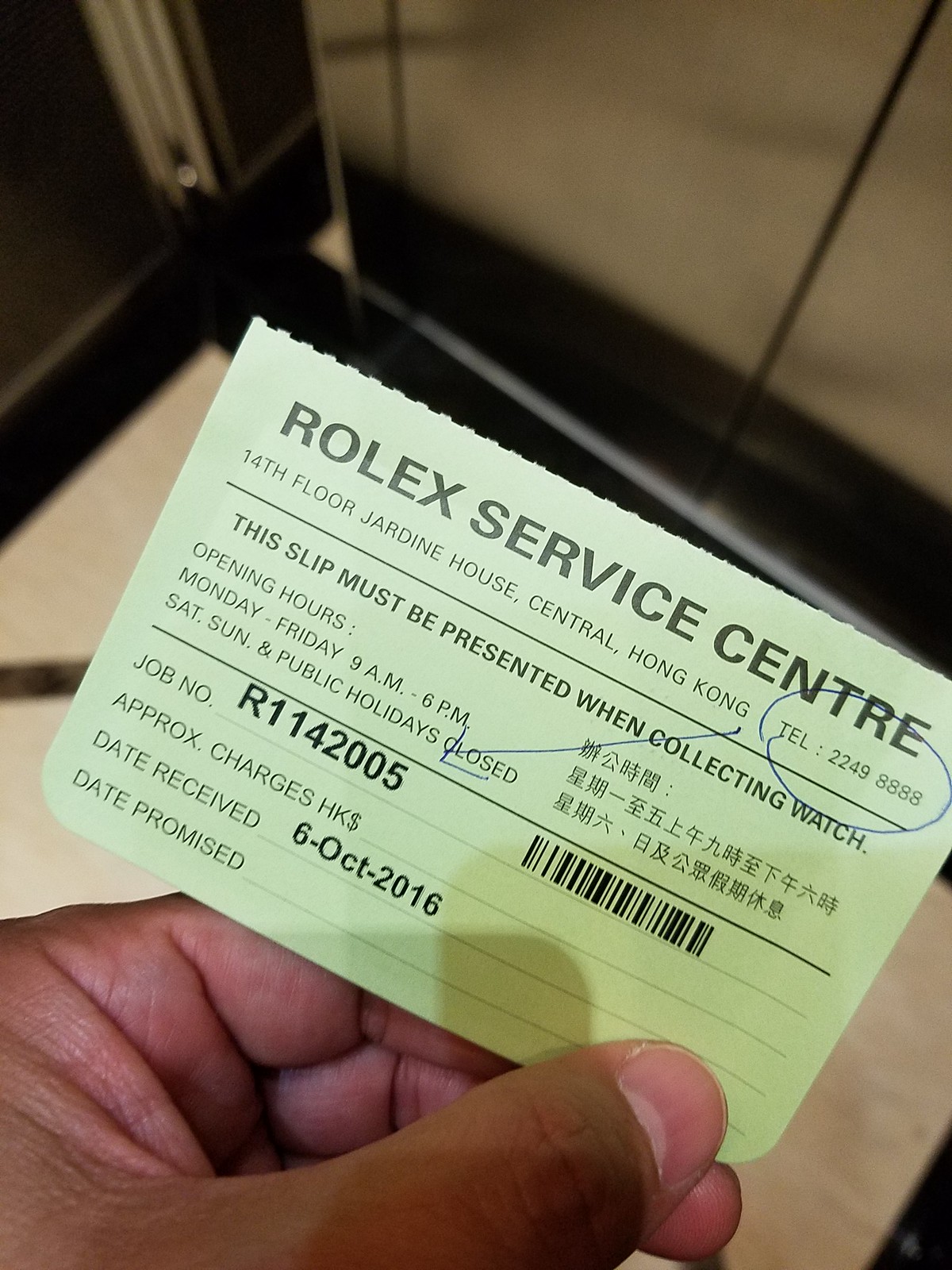The image captures a man's hand holding a detailed claim slip from the Rolex Service Center. The card, which is light green in color with visible perforation marks at the top, indicates it was torn off a larger sheet. The top section of the card prominently displays the address: "Rolex Service Center, 14th Floor, Jardine House, Central, Hong Kong," followed by the phone number "2249-8888," which is circled and connected by a blue arrow to the job number "R-114-2005" towards the bottom. The card specifies important service details: "This slip must be presented when collecting watch." The service center's business hours are listed as Monday to Friday from 9 am to 6 pm, with closures on Saturdays, Sundays, and public holidays. The card includes an area for approximate charges in Hong Kong dollars, which is left blank, and a barcode situated next to the job number. Stamped on the card is the date received, "6th October 2016," while the date promised remains unstamped. Held between the man's thumb and forefinger, the card is shown against a background that suggests an open briefcase, with the man's hand casting a shadow over the card.